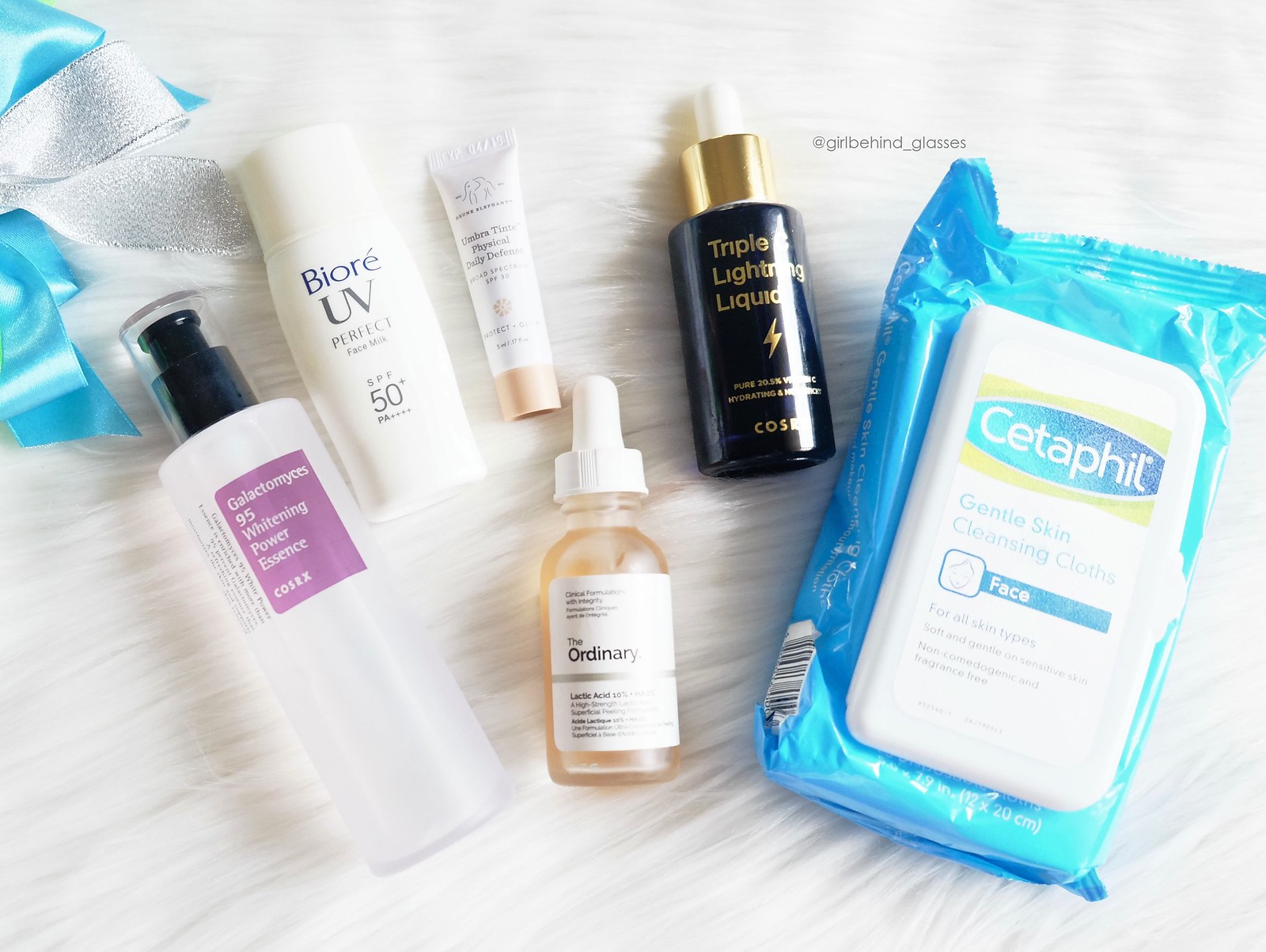This photograph showcases an elegant arrangement of beauty products laid out on a pristine white fur surface. In the upper left-hand corner, a delicate bow in a sky blue hue, intertwined with a sliver of silver glitter, adds a touch of sophistication to the scene.

The array of items includes:

1. **Cetaphil Gentle Skin Cleansing Cloths**: Packaged in a blue bag with a white, hard-top dispenser lid often seen on wipes, ensuring easy access and practicality.

2. **Triple Lightning Liquid**: Encased in a striking blue bottle equipped with a gold and white dropper top, this serum stands out with its vibrant packaging.

3. **The Ordinary Lactic Acid**: This serum is visibly peach-colored and resides in a clear bottle with a white dropper. The white label denotes its identity clearly, aligning with The Ordinary’s minimalist aesthetic.

4. **Umbra Tint Physical Daily Defense**: Presented in a small white tube featuring a peach-colored cap, this product sports an indistinguishable logo at the top, indicating its branding.

5. **Biore UV Perfect Face Milk**: Contained in a white bottle, this product emphasizes sun protection and is marked distinctly with its brand's text.

6. **Galatomides 95 Whitening Powder Essence**: This is found in a white spray bottle with a black nozzle and a clear protective cap, designed for easy application.

Adding to the visual appeal, the photograph includes a caption in the top right corner reading, “@girl behind under slashed glasses,” possibly the credit or username of the person who shared this image.